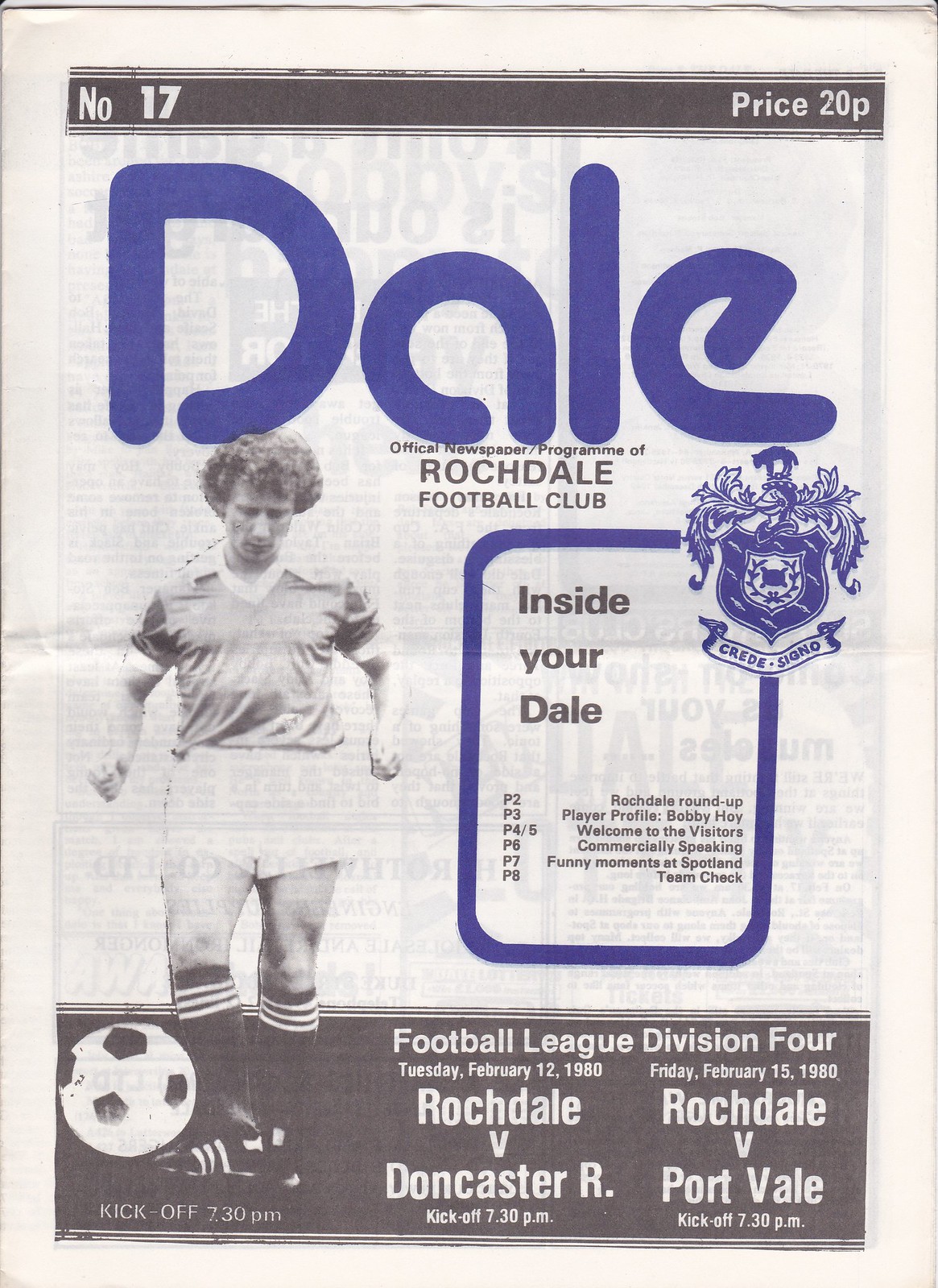This is the front cover of a vintage football club program with a clean, white background. At the top, the program features a black rectangular area with white lettering that reads "Number 17" on the left and "Price 20p" on the right. Prominently displayed in the center in large blue letters is the stylized word "Dale," with a unique font displaying missing portions at the bottom of the letters. Beneath this, in black font, it reads "Official Newspaper Program of Rochdale Football Club," with "Rochdale" spelled R-O-C-H-D-A-L-E. 

Under this title, on the left side, there is a black and white photograph of a football player mid-kick with a soccer ball. To the right of the photo, there is a rectangular blue frame that contains the text "Inside Your Dale" alongside a shield-like football club logo with additional wording.

Toward the bottom of the program, a wide black stripe spans the width of the page with white lettering detailing upcoming matches: "Football League Division 4, Tuesday, February 12, 1980, Rochdale vs. Doncaster, Kickoff 7:30 PM" followed by "Division 4, Friday, February 15, 1980, Rochdale vs. Port Vale, Kickoff 7:30 PM."